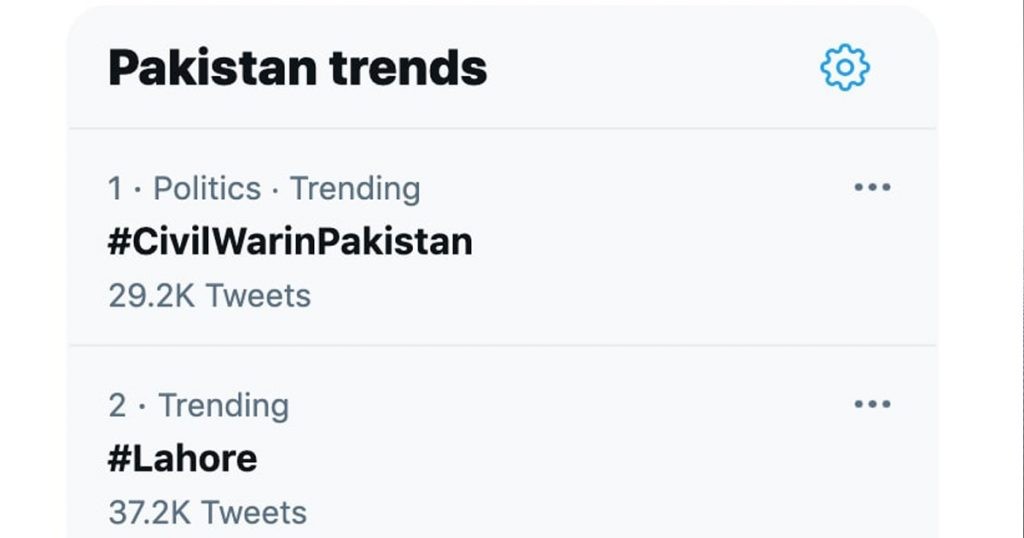The image features a settings menu labeled "Pakistan Trends," which appears to be from a phone's news widget. The top trending story is related to politics, specifically highlighting the impact of a civil war in Pakistan, tagged with the hashtag "#CivilWarImpact." This topic has garnered 29.2k tweets. Beside this trend is a context menu represented by three vertical dots. Another trending topic is "Lahore," with 37.2k tweets, also accompanied by a context menu. The layout includes a blue cogwheel icon in the upper right corner for additional settings. The background is a plain gray-white with black and gray text. The simplicity of the design leaves no further details, creating a sparse, straightforward interface.